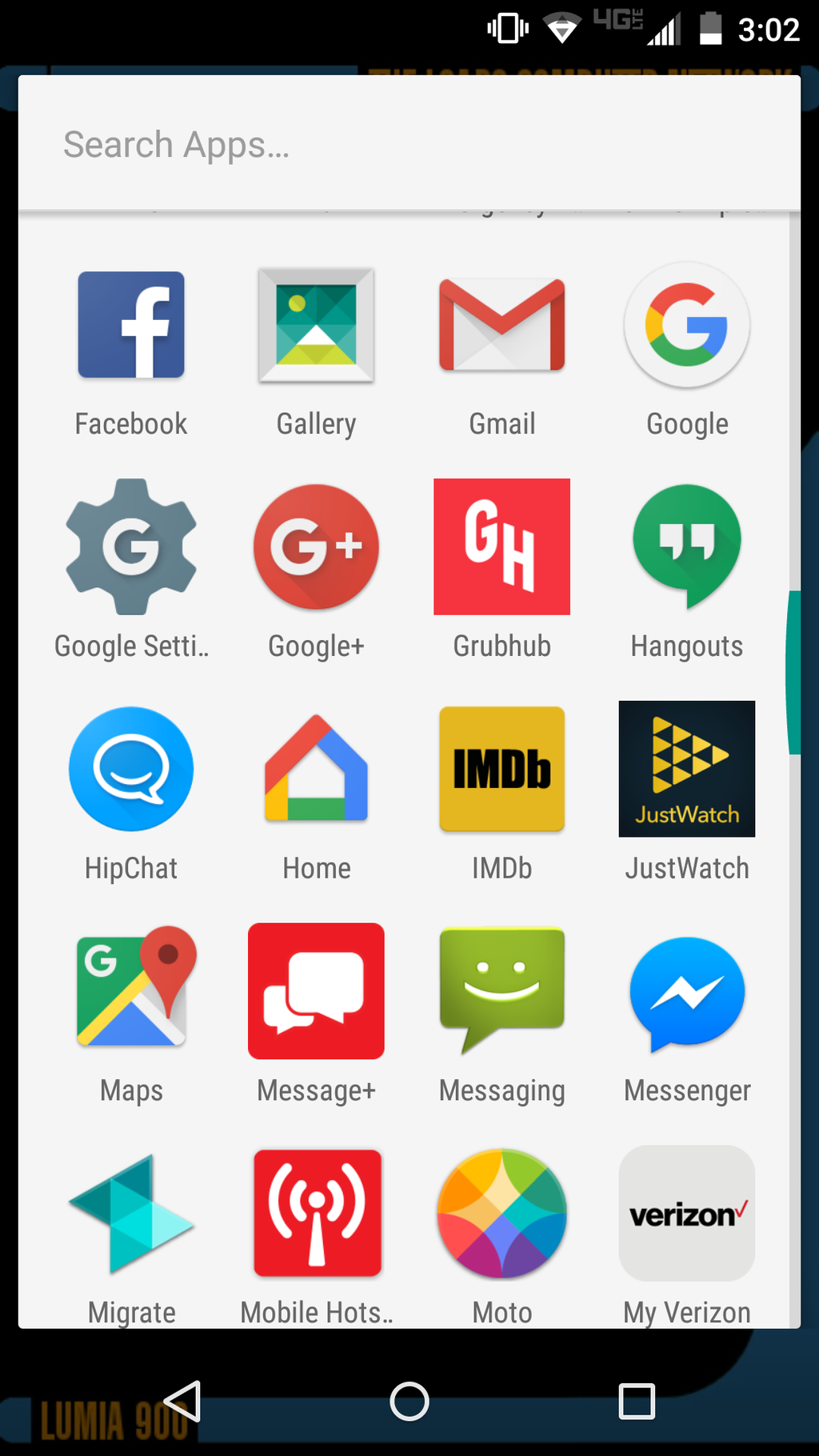This screenshot captures a detailed view of the applications page on a smartphone. On display is a pop-up window showcasing approximately 20 app icons arranged in a grid with search functionality at the top. Surrounding the pop-up, the standard phone interface is visible, including the status bar at the top showing the time and battery level, as well as navigation options at the bottom to go back home and close all apps.

The apps are presented on a white background, contrasting with the dark, black and blue tones of the phone’s usual home screen. The icons and names of the apps are clearly visible, arranged from the top left to the bottom right. The specific apps displayed include:

1. Facebook
2. Gallery
3. Gmail
4. Google
5. Google Settings
6. Google+
7. Grubhub
8. Hangouts
9. HipChat
10. Home
11. IMDB
12. Just Watch
13. Maps
14. Message+
15. Messaging
16. Messenger
17. Migrate
18. Mobile Hotspot
19. Modo
20. My Verizon

Each app icon is accompanied by its respective name, ensuring easy identification and navigation.